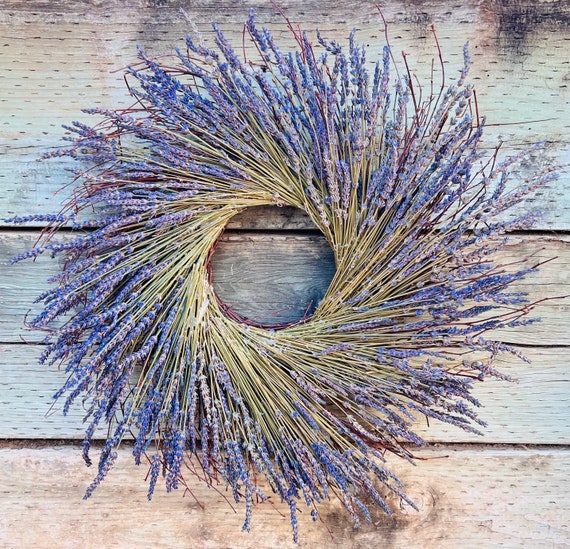The image captures a rustic, outdoor scene featuring a small wreath made from a plant that closely resembles lavender. The wreath's delicate stalks begin as a light tan color before transitioning into a vibrant green. Adorning these stems are short, bluish-purple flowers that contribute to the wreath's natural beauty. The stalks and flowers are meticulously arranged in a spiral pattern, forming a perfect circle. The wreath rests on a weathered wooden surface, characterized by uneven planks that exhibit a mix of colors—light brown, dark brown, black, and hints of blue—with visible stains and chipping paint. The wood also has black spots scattered across it, adding to the aged, rustic charm of the scene.